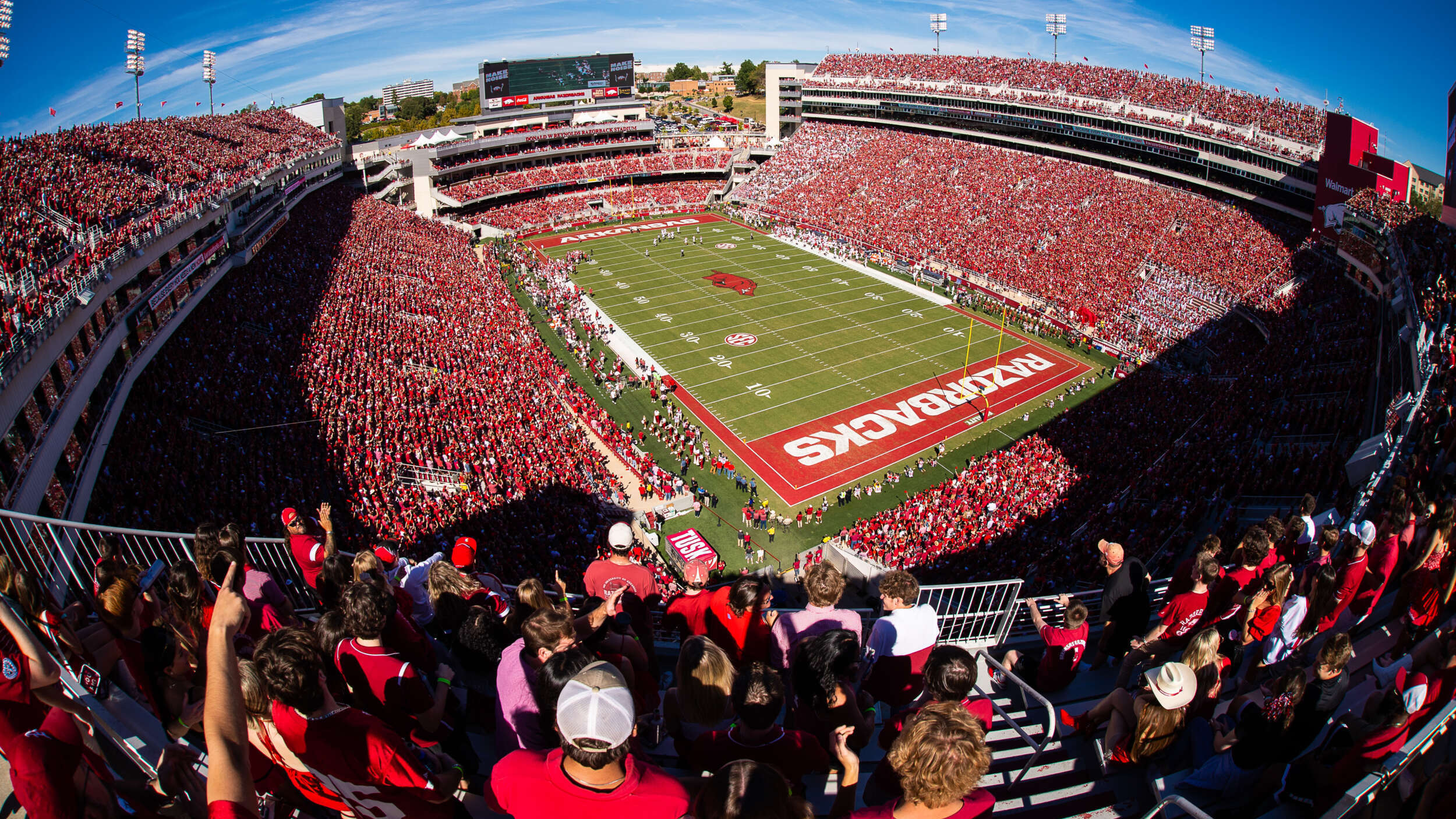An expansive, overhead, wide-angle shot captures the vibrant atmosphere of the Razorbacks football stadium during a game. The bright, sunny day highlights the intense energy as the stadium is packed with nearly 60,000 to 70,000 enthusiastic fans, predominantly wearing red and white, the team's colors. The view encompasses almost the entire stadium, with occasional shadowed areas contrasting against the brightly lit sections. The grassy football field, marked with horizontal lines counting by tens and framed by yellow goalposts, features players and coaches scattered around its outskirts, engaged in the game. Bold white letters on a red background spelling "Razorbacks" dominate both end zones. A large screen at the far end commands attention with the phrase "MAKE NOISE!" in white, while the towering stadium lights loom above. The curved quality of the image suggests it was taken with a fisheye lens, providing a visually dynamic and immersive perspective. In the foreground, fans are visibly excited, standing, clapping, pointing, and cheering, contributing to the electric atmosphere. The bright blue sky with a few scattered clouds frames the scene, underscoring the midday timing, inferred from the distinct shadow patterns across the stadium.